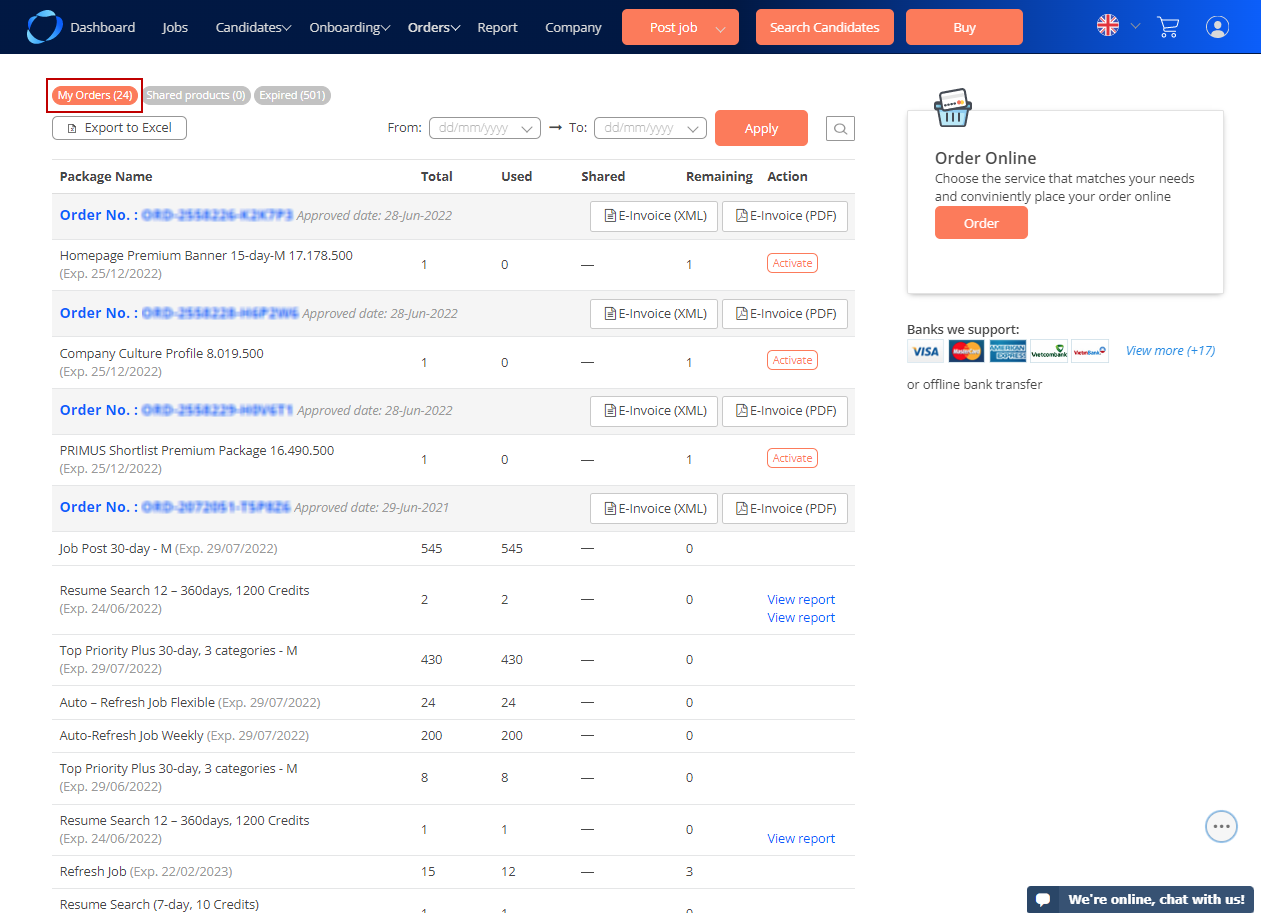This image is a screenshot of a website's dashboard interface. At the top left corner, the word “Dashboard” is prominently displayed next to a small circular logo. The main menu, situated alongside the dashboard indicator, includes options labeled as Jobs, Candidates, Onboarding, Orders, Reports, and Company.

There are three prominent buttons below the main menu, each with a gradient hue that transitions between shades of orange and pink, and white text. The buttons are identified as "Post Jobs," which features a drop-down arrow, "Search Candidates," and a simple "Buy." Adjacent to these buttons, there is a circular icon displaying a red "plus" symbol within a crew emblem, a shopping cart icon, and a profile icon.

On the left side, below the main navigation area, appears the "My Orders" section with a notification indicating a count of 24. Underneath this section, there is a list starting with the category "Order Number" and "Job Posts."